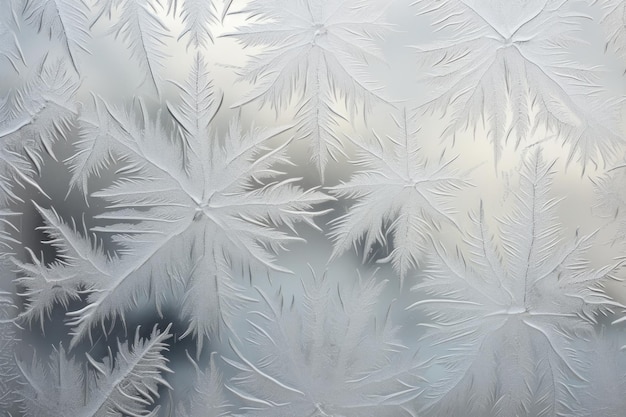The image portrays a close-up view of a glass window adorned with intricate etchings of white, wispy leaf-like shapes, possibly resembling a mix between maple leaves and feather patterns. The frosted glass features a silvery-tinted translucence, giving it a delicate, almost ethereal quality. The leaf designs, varying in shape and size, are elevated off the surface, suggesting they were either painted or sprayed on. The stems of the leaves are accentuated with slightly elevated white trimming, some of which are highlighted with hints of silver, enhancing their detailed appearance. The background behind the glass is blurred and features streaks of light gray, dark gray, and white, creating a soft, dreamy contrast to the intricate foreground. The overall effect gives the impression of looking through glass to a wintry, feathered landscape, rich with delicate patterns and subtle gradients of light and shadow.